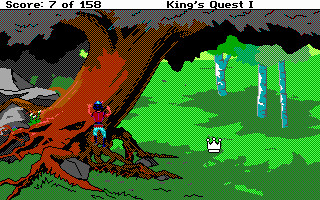This is a detailed image of a gameplay screen from King's Quest I. In the top left corner, the score is displayed as 7 out of 15 points. To the right, the game's title, "King's Quest I," is prominently shown. The taxon number is written in black text. The central focus of the image features a large tree stretching from the bottom left to the top of the frame. The trunk and branches of the tree are depicted in red and brown colors, while the leaves at the top appear gray. The ground is covered with a field of green grass. Notably, a white crown rests on the grass, situated roughly in the middle of the image. In front of the towering tree stands a person, adding a sense of scale to the scene.